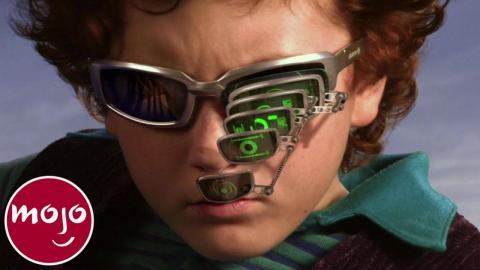The image presents a close-up shot of a young boy, roughly 8 to 15 years old, who has curly red hair cascading slightly over his ears and forehead. He wears silver glasses that prominently feature an elaborate contraption on the left lens—five smaller lenses extending outward, each with a silvery metal frame and displaying green scientific imagery. His attire includes a teal collared shirt, possibly layered over a black piece of clothing. The boy’s face, from forehead to chin, appears slightly bewildered, as if he’s examining something intently through his multi-lens setup, reminiscent of a high-tech gadget from a "Spy Kids" movie. Positioned at the lower left corner of the image is a distinctive red circular logo with a white border, bearing the inscription "Mojo". The logo creatively forms a smiley face using the letters, with the 'J' representing the nose and the two 'O's as the eyes, completed with a small smile beneath.